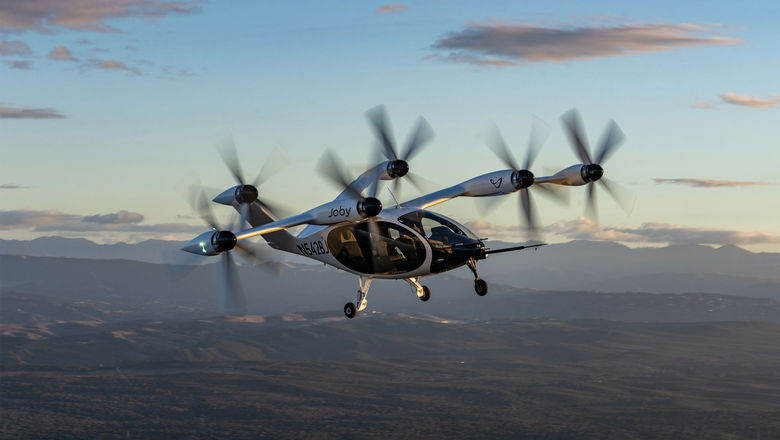The image depicts a uniquely designed, futuristic helicopter that doesn't resemble traditional models. The aircraft features multiple propeller blades, with five in the front and one at the back, all of which have black tips. The body of the helicopter, which appears to be silver and partly covered with glass, is labeled with "Joby" on one of the blades and "N5428J" towards the rear. This distinctive helicopter appears somewhat plane-like and seems to blend elements of both vehicles. It is equipped with small landing wheels, contrary to the statement of having only one wheel. The background showcases a dusk sky filled with a few dark gray clouds, with a mountainous horizon visible along with a grassy field below, giving the entire scene an expansive and serene backdrop.